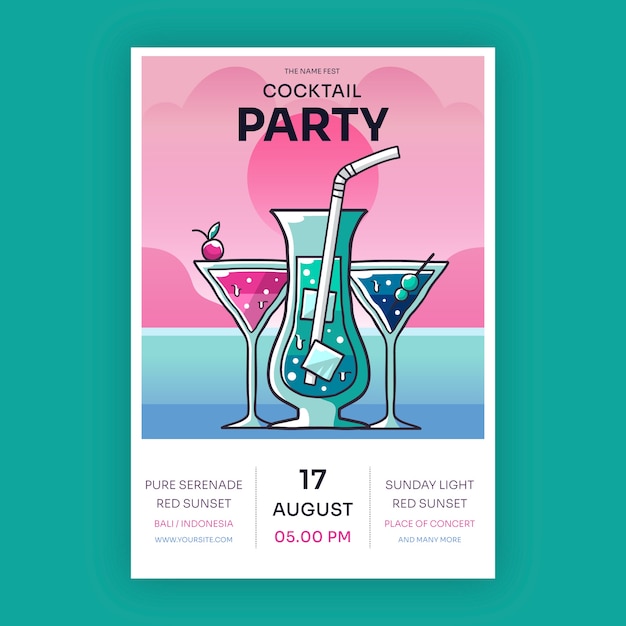This meticulously hand-drawn flyer for the Namefest Cocktail Party prominently features the event name in striking black text at the top. The main visual comprises three stylishly illustrated drinks against a playful, textured background blending hues of turquoise, purple, and pink with circular patterns. The drinks are intricately detailed: the left martini glass contains a vibrant pink liquid garnished with a cherry, the central regalés-style glass holds a bluish-green drink with two ice cubes and a straw, and the right martini glass, filled with a dark blue liquid, is adorned with skewered olives. Essential event details are elegantly arranged at the bottom, stating, "Pure Serenade Red Sunset, Bali, Indonesia," alongside the URL "www.yoursite.com." Additional information includes the date and time, "17 August, 5 p.m.," and enticing phrases like "Sunday Light, Red Sunset, Place of Concert, and many more," evoking the promise of a serene, picturesque event.